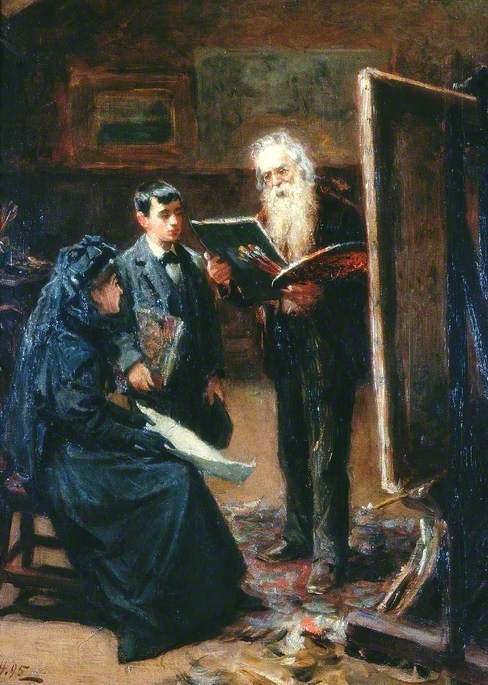In this vertically aligned rectangular painting, a striking Renaissance style unfolds in a rich, detailed composition. At the center stands an elderly man, adorned in dark, possibly black clothing, with distinguished white hair and a flowing beard. His gaze is focused intently downward at an open book held in his right hand, while his left hand grasps a round artist's palette brimming with colors and paintbrushes. Directly behind him, a large canvas looms on an easel, its surface turned away from the viewer.

To the left of the man, a young boy, appearing to be around 10 to 12 years old, stands attentively. He is dressed in a dark suit complete with a white shirt and bow tie, and holds a book in his right arm. His short, dark hair contrasts with his formal attire.

Seated next to the boy is a woman enveloped in black garments, including a long, drapey dress, black gloves, and a head covering that resembles a veil. She holds a long piece of white paper, adding a stark visual interest to her dark ensemble. Her wooden chair’s legs peek out from beneath the folds of her dress, emphasizing the setting's timelessness.

The trio is positioned within a room where the walls create a somber ambiance, blending shades of brown and black. The lower portion of the walls features dark wood paneling, while the upper half is painted in a dark hue. Adorning the walls are two indistinct paintings, their details lost in the dimly lit background. The floor beneath the artist reveals beige tones, marred by splatters of paint, suggesting this space also serves as his creative studio.